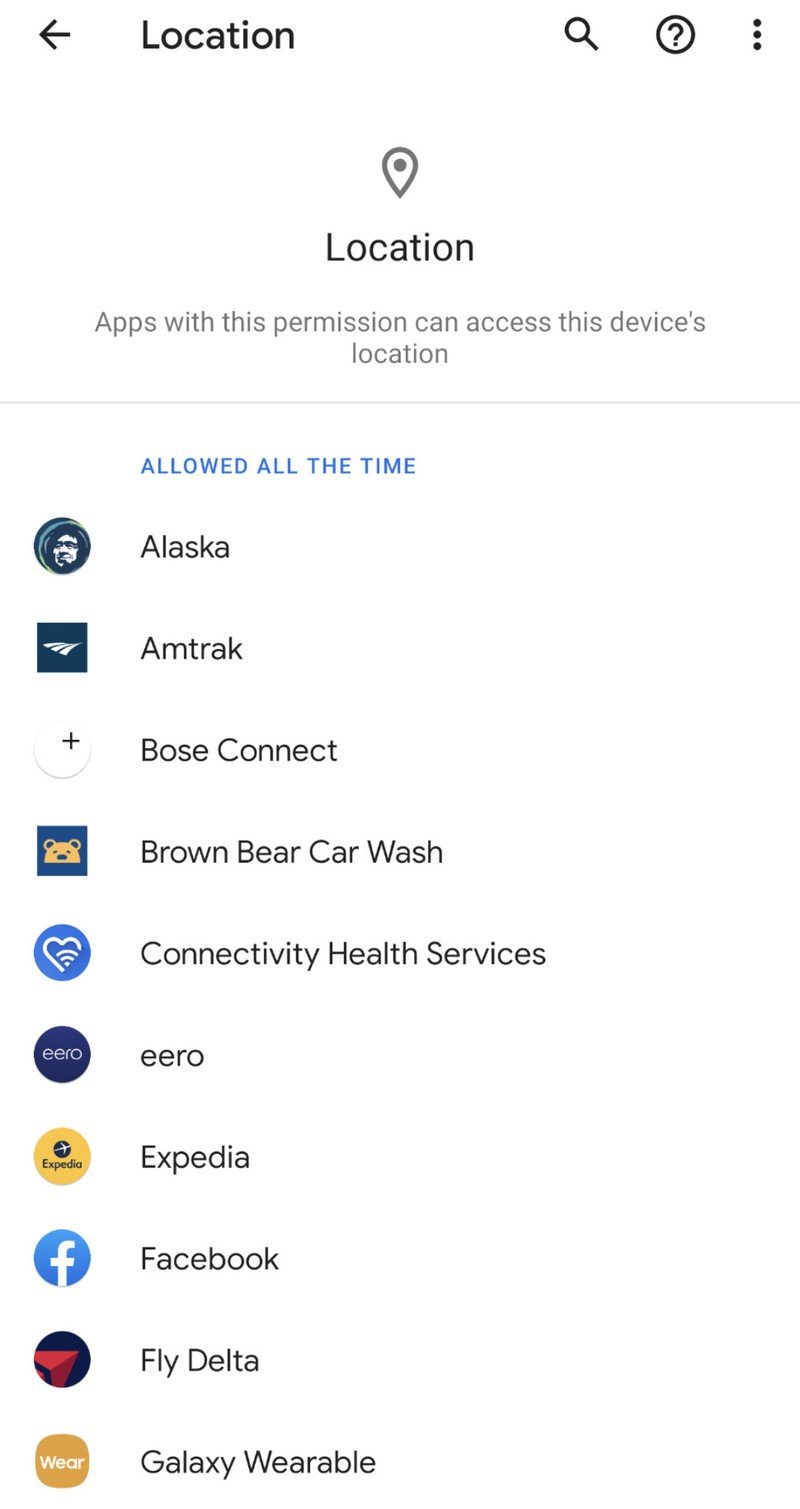The image is a screenshot from a mobile device, likely a smartphone or tablet. At the very top of the screen, there is a black header bar containing a back arrow on the far left. Next to the back arrow, the word "Location" is displayed in black letters. On the right side of this header bar are three icons laid out from left to right: a search icon, a question mark icon, and a hamburger menu icon.

Beneath the header bar, centered on the screen, is the word "Location" accompanied by a standard gray location icon to its left. Directly below, a subtitle reads: "Apps with this permission can access this device's location."

Further down, the screen lists all the apps that have location permissions under the section titled "ALLOWED ALL THE TIME," with the section title in blue capital letters. The apps are presented alphabetically, each accompanied by its corresponding icon. The list begins with "Alaska" at the top and includes "Amtrak," "BOSE Connect," "Brown Bear Car Wash," "Connectivity Health Services," "Eero," "Expedia," "Facebook," "Fly Delta," and "Galaxy Wearable."

The screenshot features a primarily white background and lacks any visible borders.